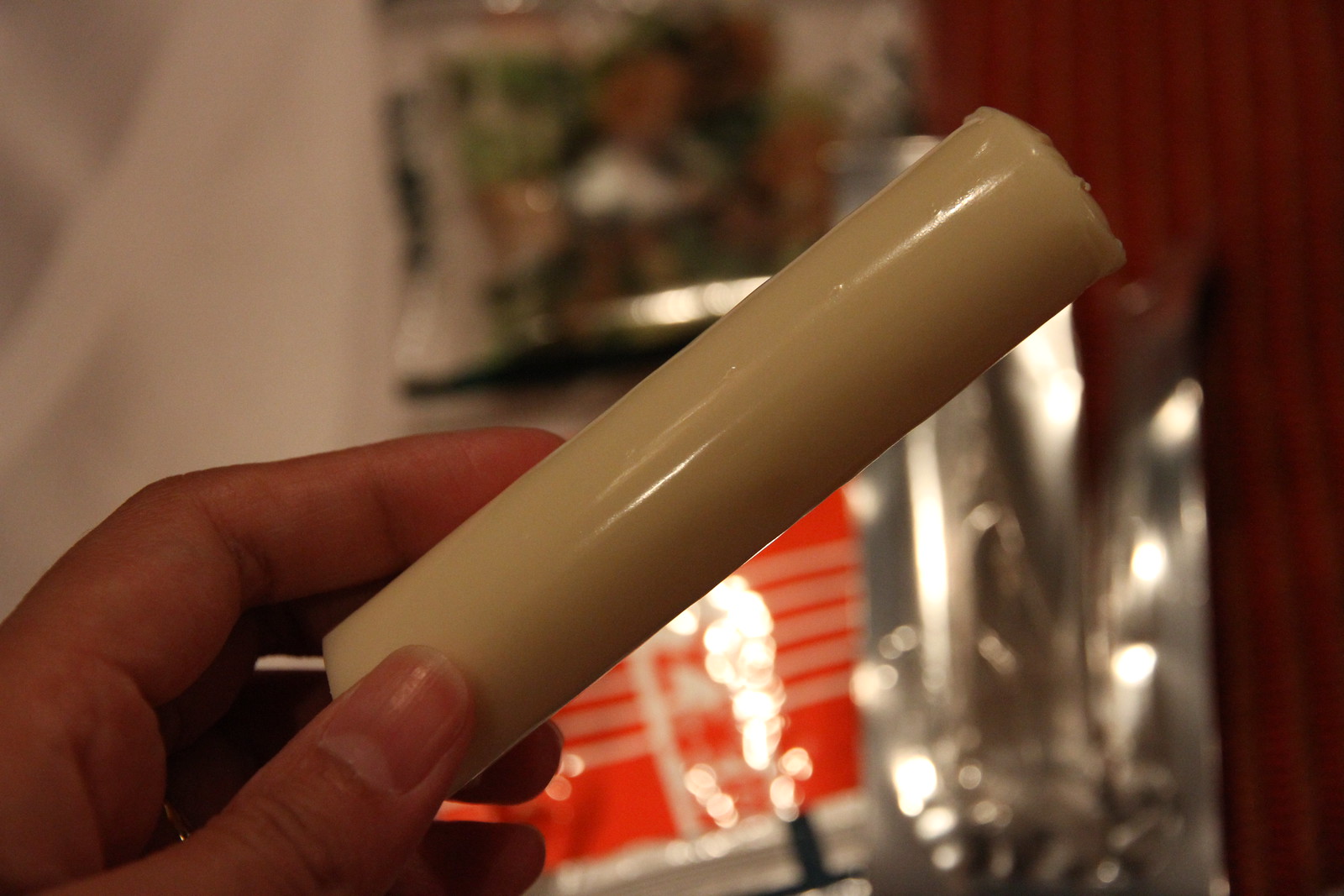A photograph depicts a zoomed-in view of a light-skinned hand, possibly male, holding a cylindrical white object diagonally from the lower left to the upper right. The hand, seen partially, showcases neatly manicured nails, with visible fingers and thumb grasping the object, which could be a candle or a cheese stick. The background is blurred, imparting an indistinct feel but with noticeable elements. On the right, there's a red fabric, possibly a curtain or material, and a glare of light. Some white lines run across this red fabric in the background. Above the cylindrical object, a mix of colors including yellow, green, dark green, and beige, possibly part of a festive or Christmas scene, adds to the haziness. There is also a metallic or glass-like object with a silver appearance. Toward the left, part of the room's white flooring is visible, juxtaposing the softer blur of the other elements.